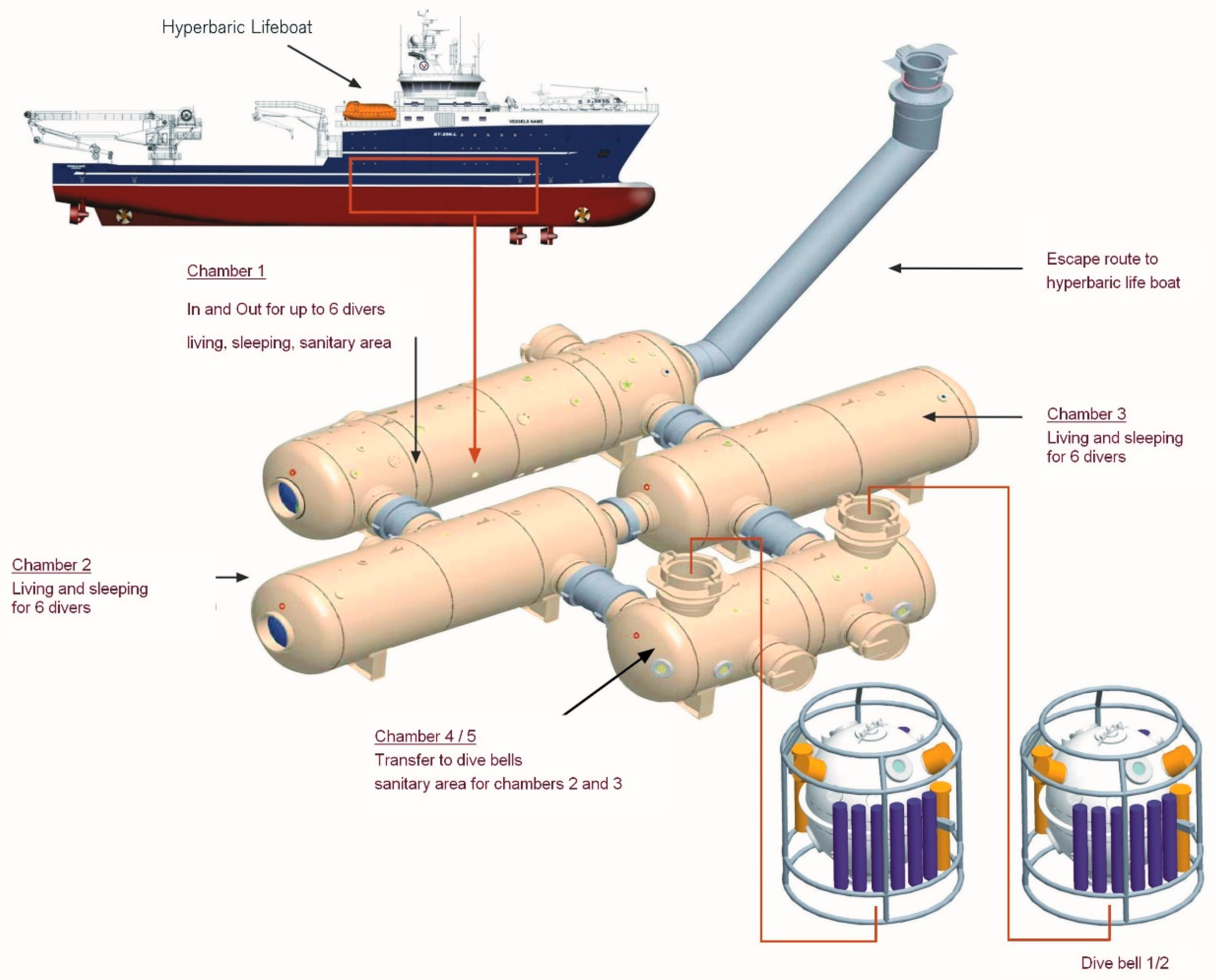This detailed diagram illustrates the structure and function of a hyperbaric lifeboat aboard a large ship, emphasizing its use for diving crews to maintain stable pressure levels. The lifeboat is highlighted in its position on the vessel, accompanied by a comprehensive breakdown below. The escape route is indicated by a pipe, likely designed for swift evacuation. The interior layout features four main chambers with specific purposes:

1. Chamber One: Accommodates up to six divers, functioning as a living, sleeping, and sanitary area.
2. Chamber Two: Provides living and sleeping space for another six divers.
3. Chamber Three: Similarly, this chamber houses six divers, offering living and sleeping facilities.
4. Chambers Four/Five: Includes sanitary facilities for Chambers Two and Three and allows transfer to the dive bells.

The diagram also shows two dive bells, essential for divers to descend deeper into the ocean. This setup enables divers to re-enter the ship without decompressing after each dive, thereby preventing decompression sickness. The lifeboat's intricate design underscores its primary function: ensuring the safety and well-being of the crew in hyperbaric conditions.